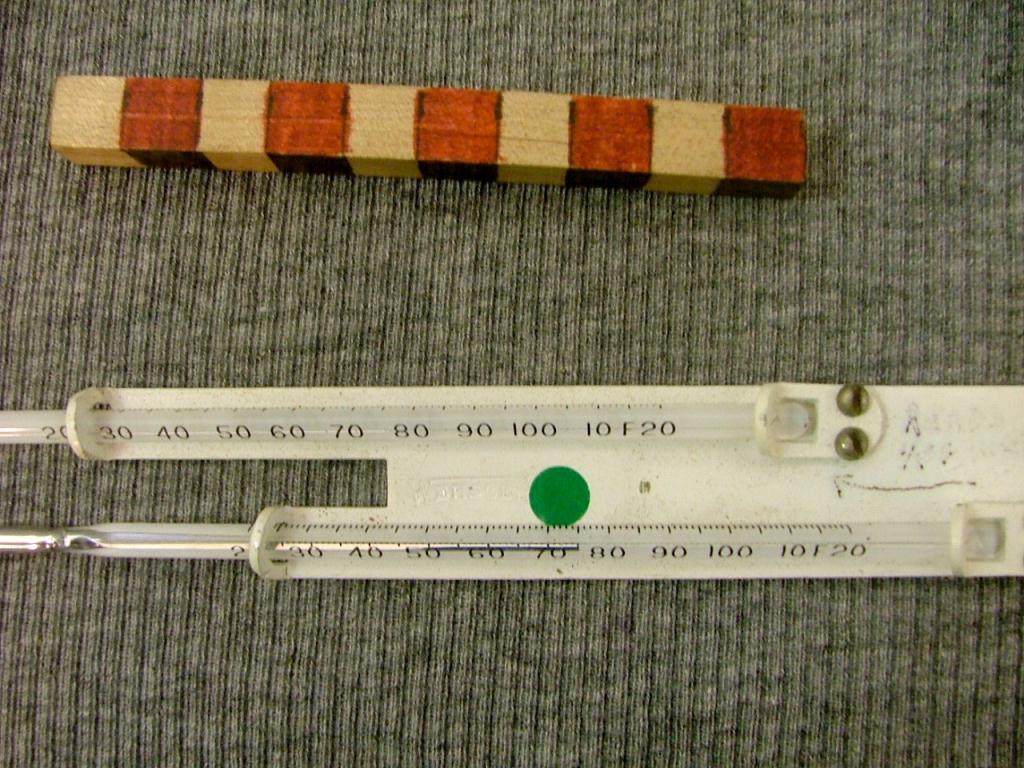At first glance, the image appears to show two thermometers, which could either be wall-mounted or oral thermometers, though it's not entirely clear. They are placed horizontally on a dark gray fabric with a vertical grain texture. These thermometers are attached to a singular piece of white metal. In the top portion of the photograph, there is a square dowel marked with a checkered pattern, featuring alternating brown and white boxes, drawn to create a contrasting design.